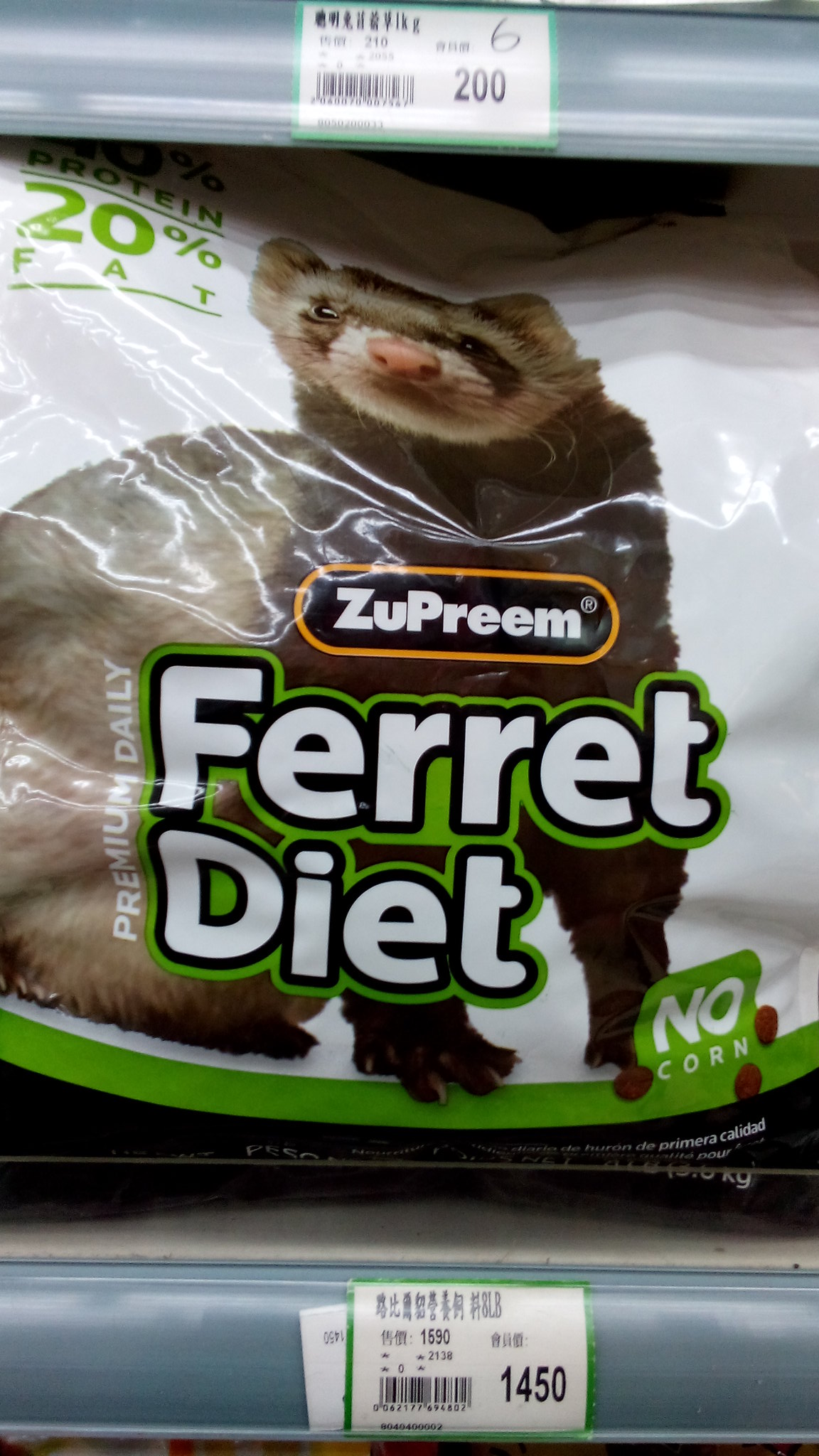"Photograph of a bag of ferret feed from the brand Zuprin™. The bag is clearly labeled as 'Zuprin Premium Daily Ferret Diet' and highlights that it contains 'No Corn'. It boasts a nutritional profile of 'Protein with 20% Fat'. The packaging features an appealing image of a ferret looking directly at the camera, as if to suggest its approval of the product. The ferret appears to be sitting sideways, casting a charming gaze towards the potential buyer. At the bottom of the bag, an illustration displays the ferret food, which resembles small cocoa puff-like pellets. The bag is placed on a shelf with a barcode marked '14-1500' and some additional, unreadable lettering, against a light blue, slate blue-colored shelf edge."